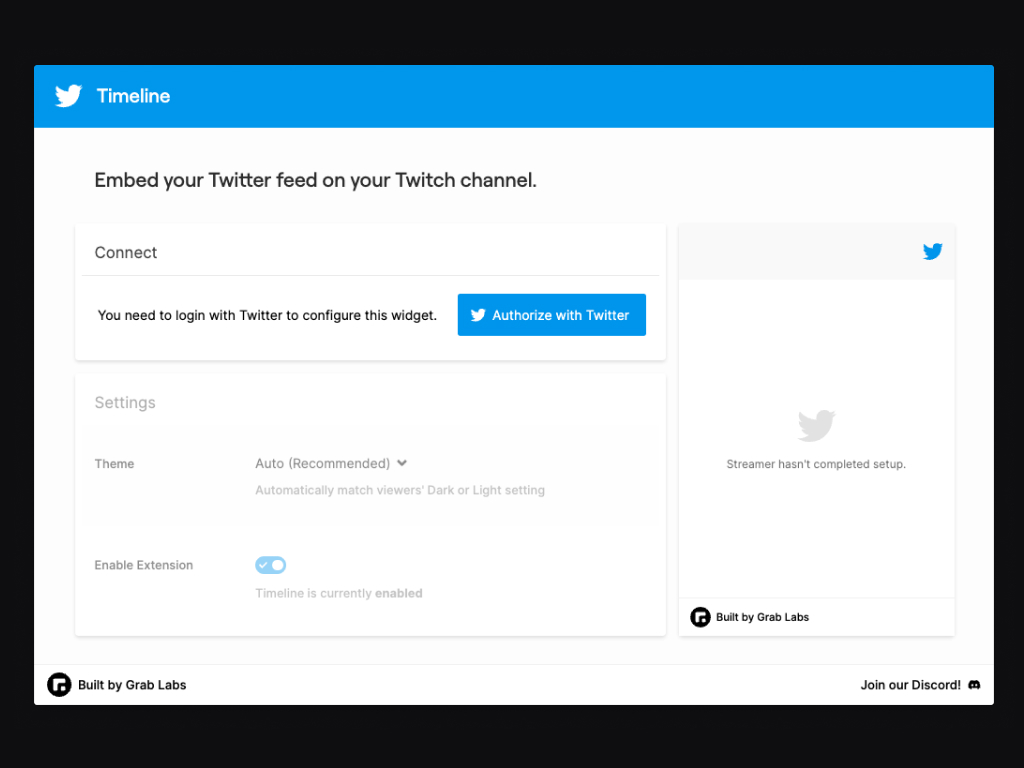The image features a rectangular interface with a black border surrounding it. Across the top, there is a blue banner showcasing a white Twitter bird icon alongside the word "Timeline" in white text. Beneath this banner, the remaining portion of the image is predominantly white.

The text below the banner reads: "Embed your Twitter feed on your Twitch channel." Following this is a blue button that contains white text, instructing users to "Authorize with Twitter" and depicting a small white Twitter bird icon. To proceed with the configuration, users need to log in with their Twitter account.

Further down, the image displays a grayed-out section with settings options. It includes an option labeled "Settings, Theme," which features a dropdown menu for "Auto-recommend" and a note explaining that it will "Automatically match viewer's dark or light setting." Below this section is an "Enable Extension" feature, indicated by a selected radio button and a note stating "Timeline is currently enabled."

On the right side of the image, there is an additional small box featuring the blue Twitter bird and a message informing users that "Streamr hasn't completed setup." Near the bottom, the text "built by Grab Labs" appears in black, followed by a final footer where "built by Grab Labs" is reiterated on the left. On the right side of this footer, there is an invitation to "join our Discord."